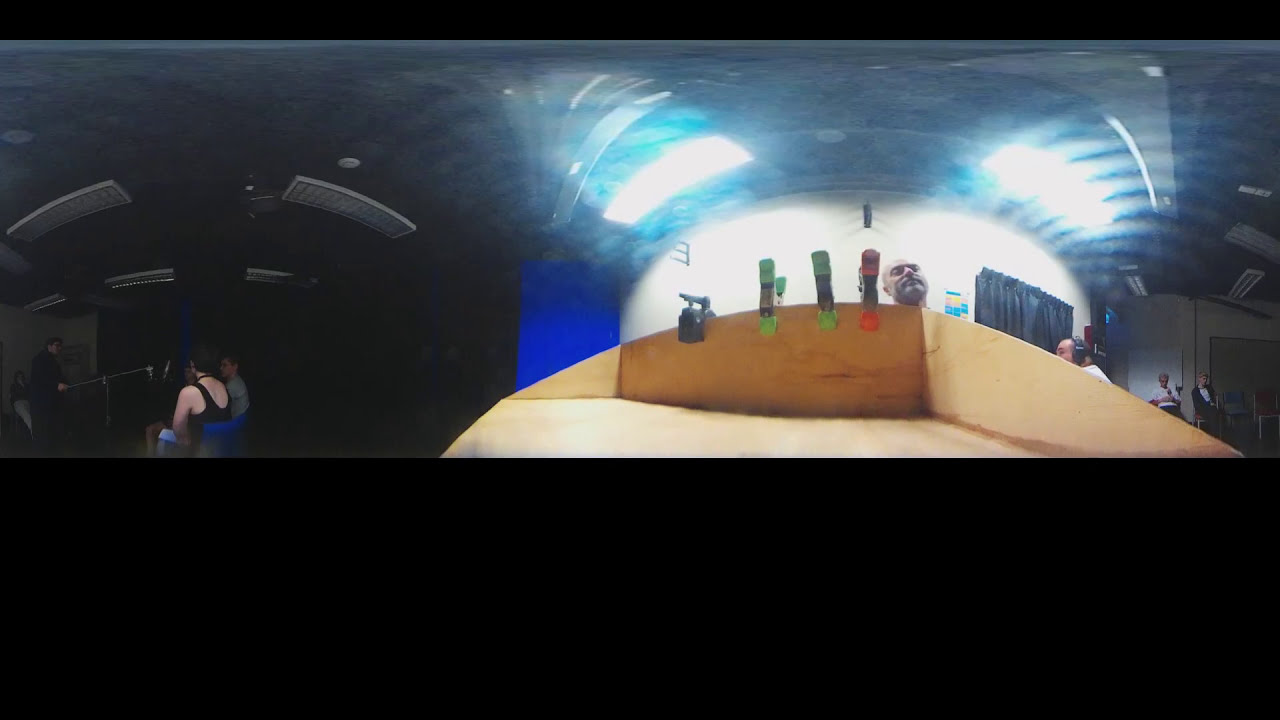In the image, we observe an indoor setting that appears to be a warehouse, characterized by a mixture of natural and artificial lighting. The central focus is a wooden desk with a rounded top located on the lower right side. On the desk are several metallic clips, commonly used for securing items, with two featuring green rubberized grips and one with a red grip.

Peeking over the side of the desk is a bald man with light beard stubble. To his right, another individual wearing headphones and a white shirt is partially visible. Behind them, two more people are sitting, one in a white shirt and the other in a black and white outfit. Specifically, towards the left side of the image, the lighting dims significantly, revealing two more people, one discernible by a t-shirt, while the other remains indistinct.

A prominent curved light feature occupies the center of the image, adding to the warehouse-like ambiance. The framing of the picture itself includes a thick black border at the bottom and a thinner black border at the top. Various colors such as black, tan, green, red, light blue, dark blue, silver, and gray are discernible throughout the scene. The spread of objects and people, none of which are centered, underscores a casual, possibly work-related environment.